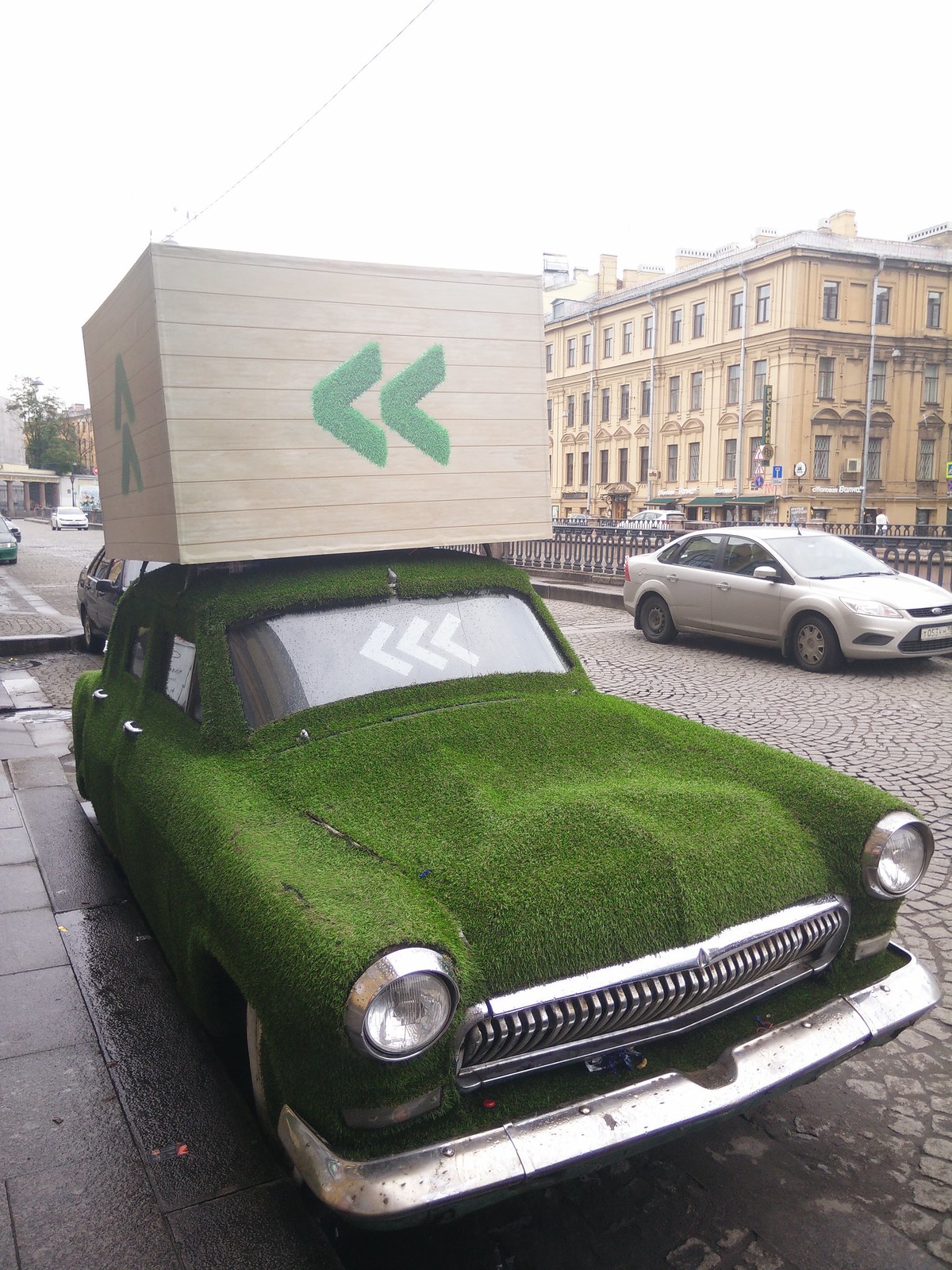This vertically aligned rectangular photograph captures a city street scene, likely in a European city with traditional cobblestone streets and a distinct old-world atmosphere. The central focus is an unusual, old-style car parked at the curb. This car stands out due to its intriguing exterior, which is entirely covered in what appears to be short, vibrant green grass instead of standard paint. It features silver-rimmed headlights, a long silver bumper, and an overall vintage design.

On the windshield, three white chevron arrows pointing left are prominently displayed against a gray background. Atop the car, a large, light-colored wooden crate sits on the roof, adorned with green sideway V's (also chevron arrows) pointing left, reminiscent of the grassy texture on the car itself.

In the background, a four-story tan stone building with numerous rectangular windows stretches upward, reaching towards a white sky. A power line crosses the top of the image, adding to the urban setting. Additionally, a small silver four-door sedan drives down the street to the right of the grassy car. Notably, the street is delineated by a walkway paved with elongated paver stones on the left side, further enhancing the scene's charming, perhaps quaint, city vibe.